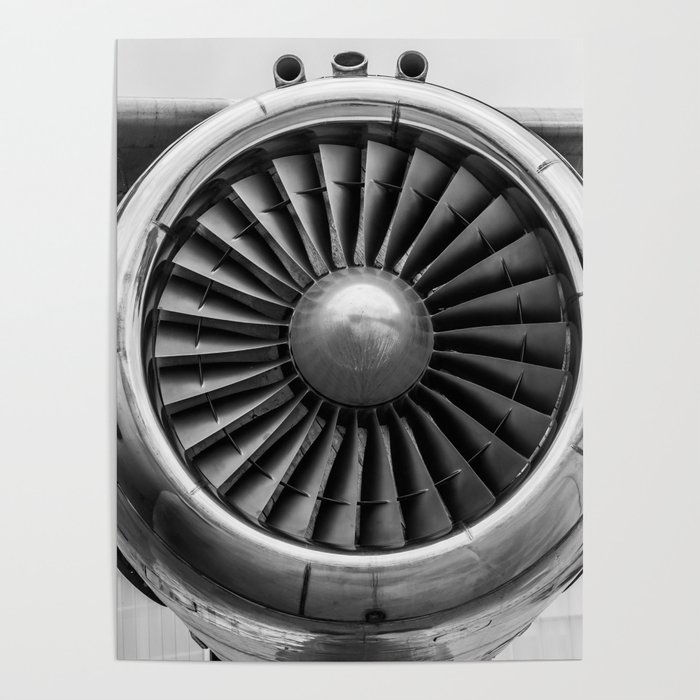This black and white photograph, seemingly an artistic print suitable for home decor, captures a close-up view of a vintage aircraft engine, likely the intake of a jet or propeller plane. The image is dominated by the engine’s circular structure, showcasing approximately 30 angled, metal fan blades surrounding a smooth, dome-like center cone, which all appear in various shades of gray and silver. The engine cowling is polished, giving it a sleek, stainless steel appearance. Notable details include three circular inlets situated on the top of the cowling, adding an element of intrigue. The scene suggests outdoor daylight conditions, with subtle hints of the engine’s mounting to the aircraft wing visible at the top. The photo's detailed texture and intricate design elements highlight the vintage machinery's robust and enduring craftsmanship, making it a striking piece of mechanical art.